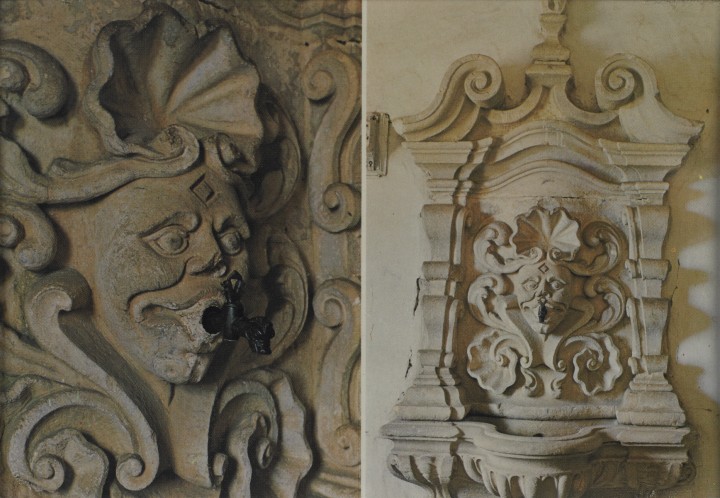The image features two side-by-side photos showcasing an old, intricately sculpted fountain attached to a white concrete wall. The focal point of the fountain is a human-like face, centered with large eyes and a diamond-shaped insignia on its forehead. Emerging from the mouth of this face is a metal spigot with a knob on top, painted black. Surrounding the face is elaborate filigree, including geometric patterns and curvilinear designs, with some elements resembling a fanned-out seashell or clamshell at the top of the head. Flanking the face are sculpted columns leading up to an archway. Below the face is a stone basin, akin to a sink, which completes the fountain structure. The sculpture shows signs of aging, including blackened and scratched areas, indicating it hasn't been restored. The overall design and detailed craftsmanship suggest that the piece is not only functional but also a work of art.